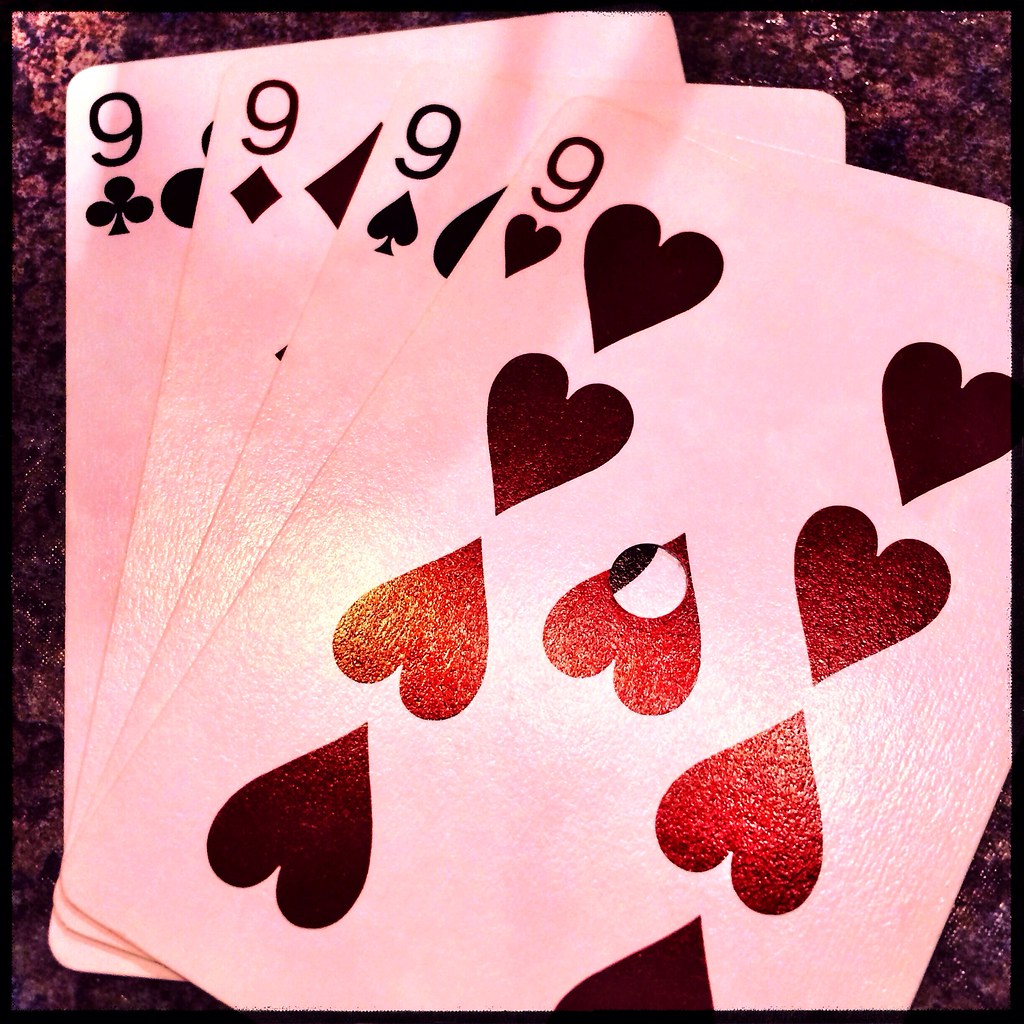The image showcases four playing cards, all featuring the number nine. The cards are arranged in a row from left to right as follows: the nine of clubs, the nine of diamonds, the nine of spades, and the nine of hearts. The nine of hearts, placed at the front, has a distinct hole in its center, cutting through one of the black hearts. 

The cards dominate the frame, with the intricate designs of the hearts on the nine of hearts drawing particular attention. The hearts on this card are arranged with two pointing up and two down on the left side, and two pointing up and two down on the right side, with a central heart situated between the two in the center column. The hole is slightly off-center, positioned a bit above and to the left.

The background appears to be a textured surface, possibly a piece of carpeting or a tablecloth adorned with tiny beads or shiny strands. The glare on the nine of hearts adds a reddish tint to some of the hearts, distinguishing them from the uniformly black hearts on the other cards.